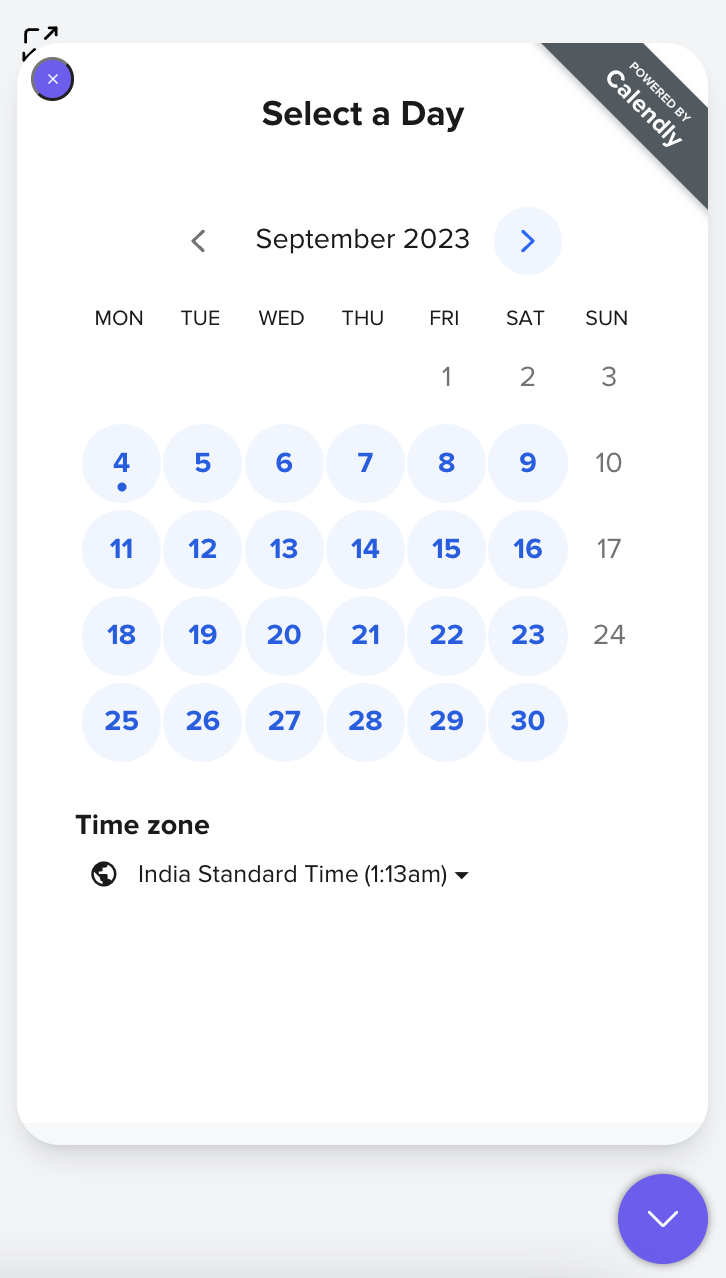The image features a gray background with multiple layered elements. In the upper-left corner, there is a small black square containing a line or arrow that extends to both the upper right and bottom left. This black square is overlaid by a white square, inside which, in the upper-left corner, is a blue-black circle with a blue interior and a white "X" at its center.

Prominently in the center of the image is the phrase "SELECT TODAY" written in black text. Adjacent to this, on the right-hand side, there is a horizontal banner in an off-gray color that prominently displays "Powered by Calendly" in white text.

Below this, there is a section featuring navigational arrows: to the left, a gray arrow points left accompanied by the date "September 23" in gray text; to the right, a highlighted light blue arrow points right. The calendar grid itself spans Monday through Sunday, with the month beginning on a Friday and ending on the 30th. The dates 1st, 2nd, and 3rd, along with the 10th, 17th, and 24th, are white with gray text, while the rest of the dates are circled in blue with darker blue numbers. Notably, the 4th has a small dot underneath it.

On the right-hand side, just below the main section, it reads "Time Zone" in black, followed by a small globe icon and "India Standard Time 1:13 AM," accompanied by a dropdown indicator. Finally, in the bottom right corner, there is a blue circle with a white down arrow inside it.